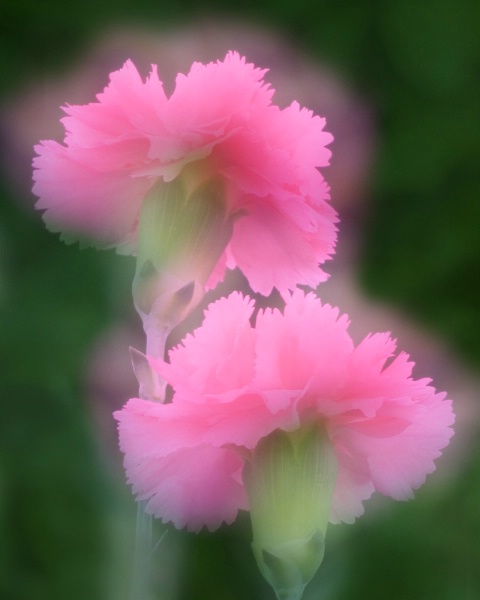The image features two light pink carnations set against a dark green background, with the corners of the frame intensifying in darkness, particularly at the top right. The flowers are positioned almost vertically, one above the other, and both are facing away, their petals displaying a delicate ripple along their edges. A dream-like, ethereal quality permeates the scene, with the carnations appearing to emit a subtle, glowing aura. This creates a soft, fuzzy white-purple halo around the petals, giving the impression they are gently illuminating the space. The stems, slightly visible but blending seamlessly into the green backdrop, occasionally reveal tiny green buds and a leaf. The composition as a whole is heavily blurred, enhancing its otherworldly, almost mystical aesthetic.